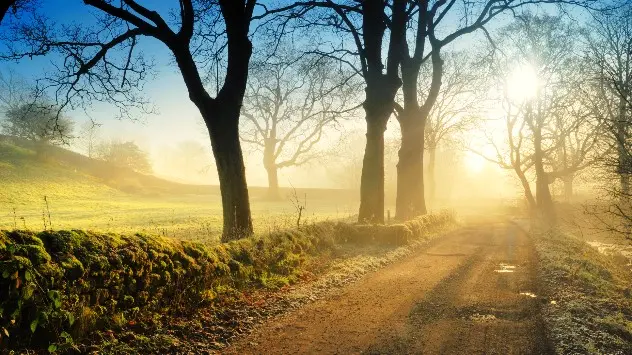The photograph captures a serene, early morning scene along a dusty dirt road. The road is centrally positioned, with large bare trees lining both its sides. A thick cloud of dust hangs in the air, illuminated by the golden rays of the morning sun that penetrate between the tree trunks. To the left of the road, the terrain slopes uphill, covered in lush green grass. In the same direction, a small stone wall separates the dirt path from an adjacent field that contains a couple of additional trees. The right side of the road shows a lower pile of dirt and scattered puddles, remnants of a recent rain that add to the tranquil atmosphere of the scene. The photograph boasts vibrant colors, with the brown dirt road and trees contrasting sharply with the green grass and leaves on some trees to the left. Though the dust obscures much of the air, the overall image evokes a peaceful, almost nostalgic feeling, making it easy to imagine taking a calm morning walk along this path.